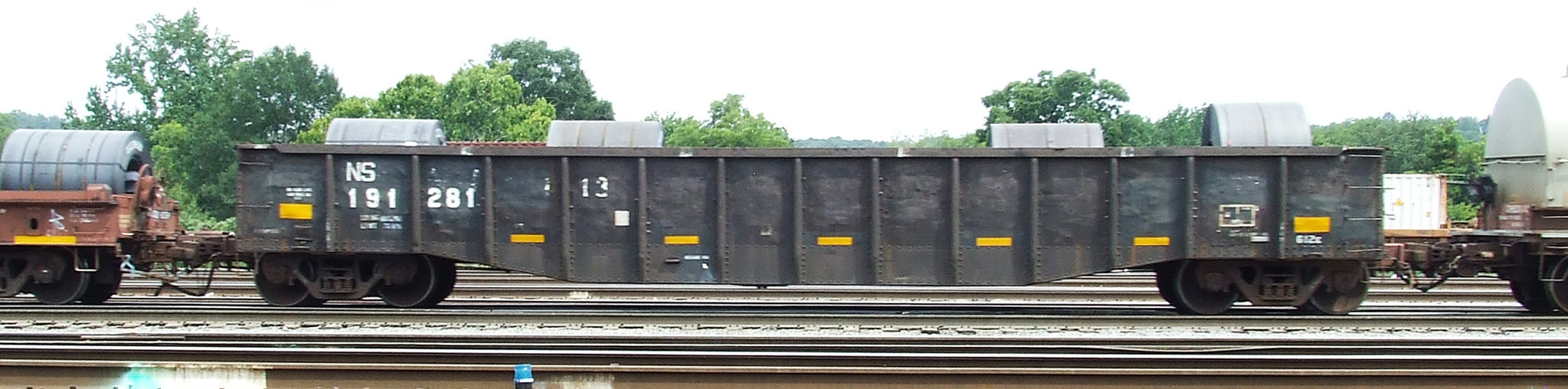The image depicts a Norfolk Southern flatbed railcar, numbered 191281, prominently placed in the center. The railcar is carrying four large, silver metal coils, two on each side. Above the number 191, the letters "NS" are painted in white. The car features black metal bars, yellow reflective lights, and a small ladder with four rungs on the side. Behind it, there is a rusty brown flatbed car also loaded with similar metal coils. At the front, another flatbed car is visible, housing a large horizontal white cylinder. The scene is set in a rail yard, with multiple tracks and a backdrop of trees showcasing varying shades of green leaves beneath a clear blue sky. The image is wide, approximately three times its height, emphasizing the length of the train and its surroundings.